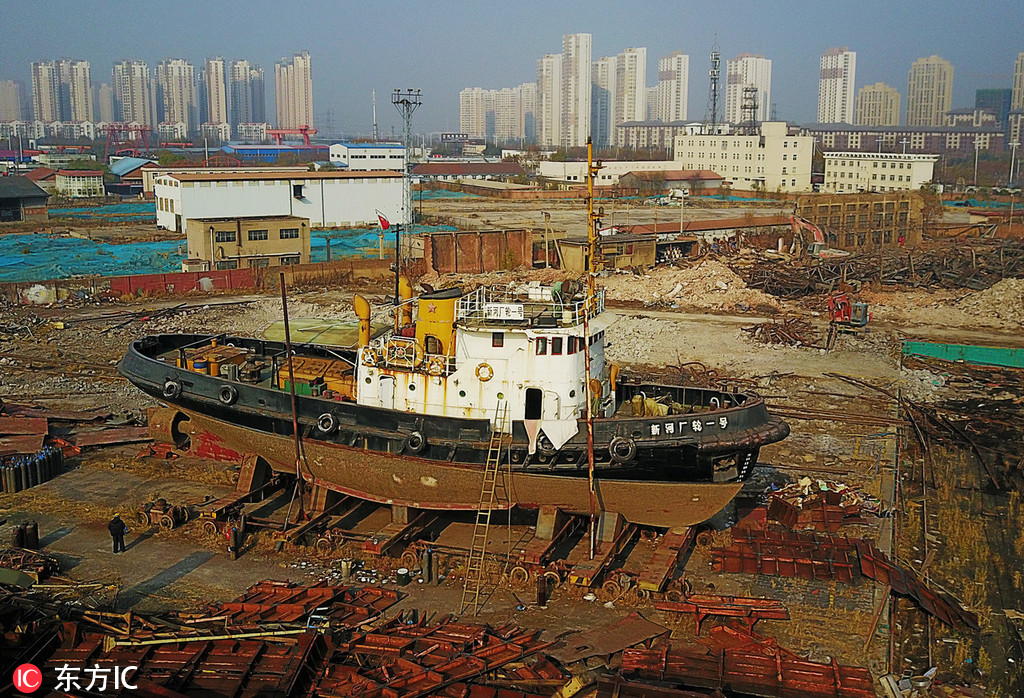The picture features an expansive, rusted shipyard bustling with activity and the signs of ongoing work. In the foreground, distant figures engage in ship repairs. Dominating the center of the image is an unfinished wooden tugboat or steamboat, supported by blocks and accessed by a ladder. The boat prominently displays Asian text, suggesting a location in East Asia, possibly China, Japan, or Korea. Surrounding the vessel are piles of scrap metal and various materials, contributing to the shipyard's industrious atmosphere. The background reveals a striking skyline of tall, old-looking skyscrapers, with high-rise residential buildings characterized by a white, monotonous appearance. The ground near a warehouse has a light blue hue, hinting at water presence. The image appears artificially enhanced with vibrant colors. At the bottom left, a logo depicting "IC" alongside Chinese characters further situates the scene in an Asian context.